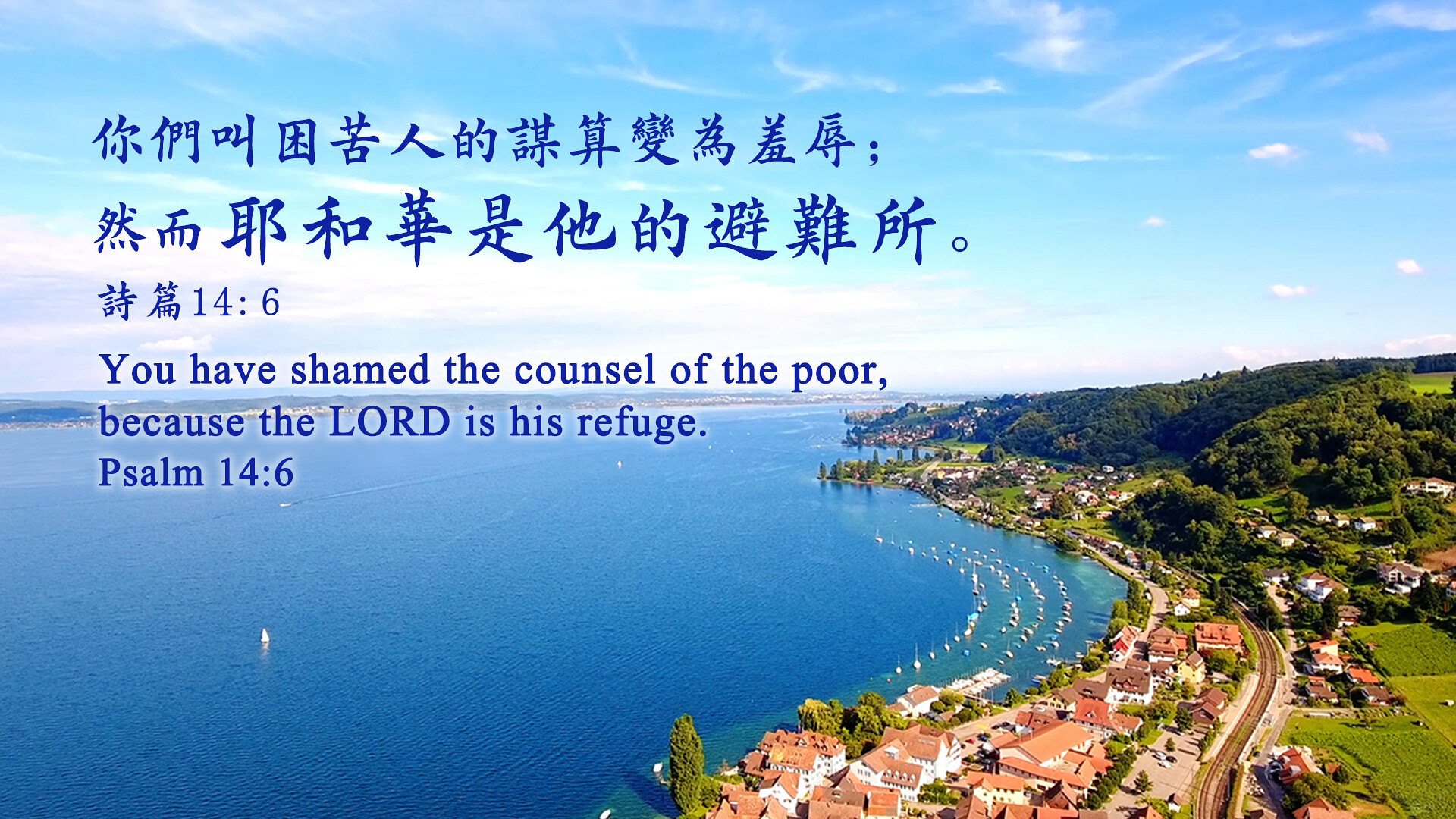This aerial image resembles a picturesque postcard of a beautiful coastal area. On the right side of the photo, there is a vast, serene body of water, which could be a big lake, part of a sea, or a bay. The water is a striking blue, and towards the middle, a lone sailboat navigates its expanse. Closer to the shore, there are four curved rows possibly comprising either beach breaks or boats, likely forming a marina. The coastline on the left is lined with houses that have distinct peach-colored roofs. Below these, there is a thin road visible amidst the land area. In the foreground, a couple of rows of houses with red roofs are positioned, while in the background, lush, green tree-lined hills rise, enhancing the natural beauty of the scenery. The upper half of the photo is dominated by a blue sky with scattered white clouds. On the horizon, another shore is faintly visible in the distance. Additionally, the image is overlaid with text; the top in Chinese and an English translation beneath it, reading, "You have shamed the counsel of the poor, because the Lord is his refuge. Psalm 14:6." The text is in a dark blue font with a subtle white glow for readability.